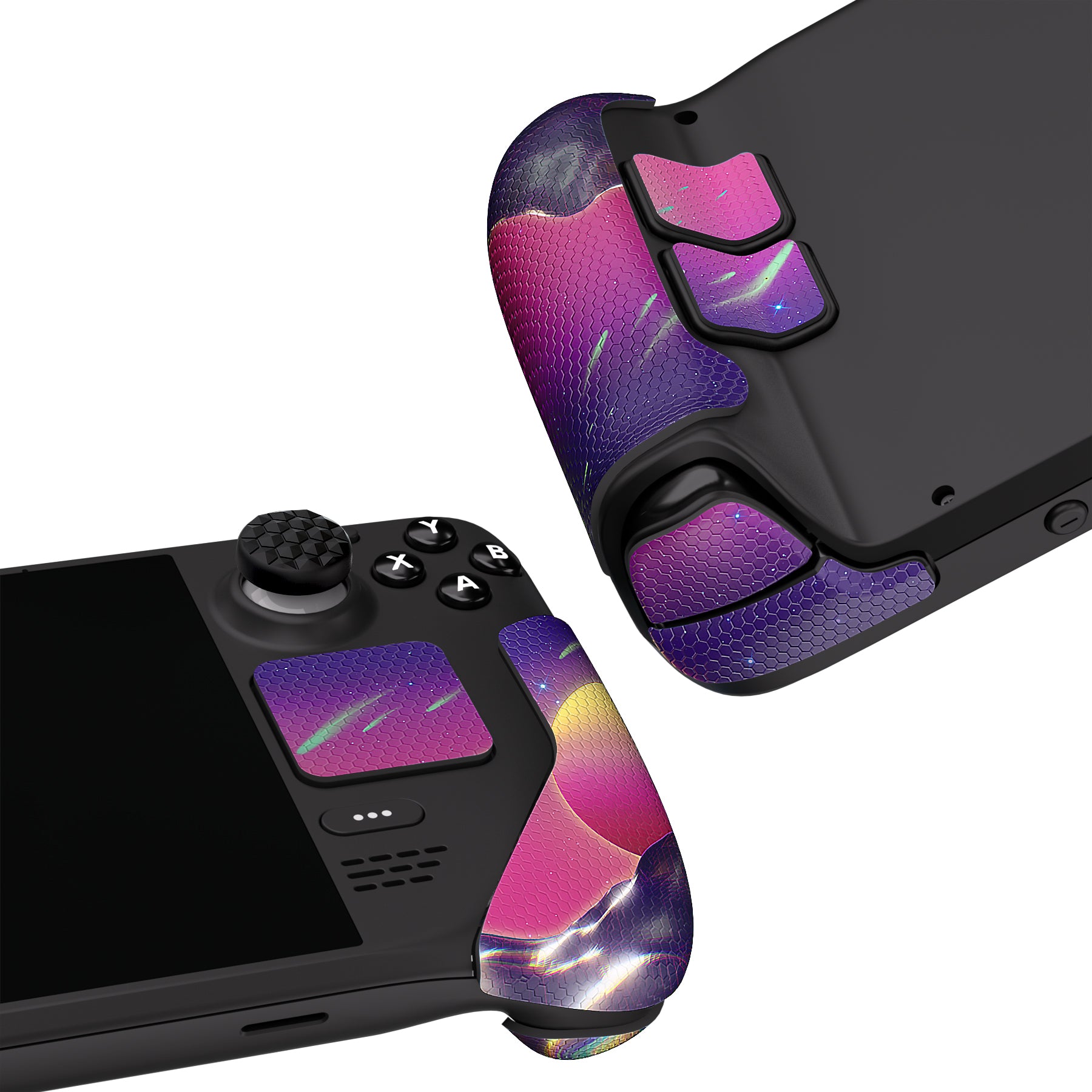The image showcases a highly detailed and realistic photograph, possibly digitally animated or edited, of a black handheld video game device similar to a Nintendo Switch. Set against a white background, the device features a sleek black frame with matching black buttons and screen. The design exhibits a distinct cosmic theme with glowing purple-pink hues on its touchpad and some buttons, as well as the handles. This cosmic motif includes elements like black-purple mountains, shining celestial bodies, green shooting stars, and comet-like streaks of yellow and white stars, creating a captivating space-like effect. The controller highlights an array of buttons marked Y, X, A, and B, alongside a directional pad designed for thumb use. The photograph presents both the top and bottom views of the controller, revealing additional finger rests on the back for a comfortable grip during gameplay.